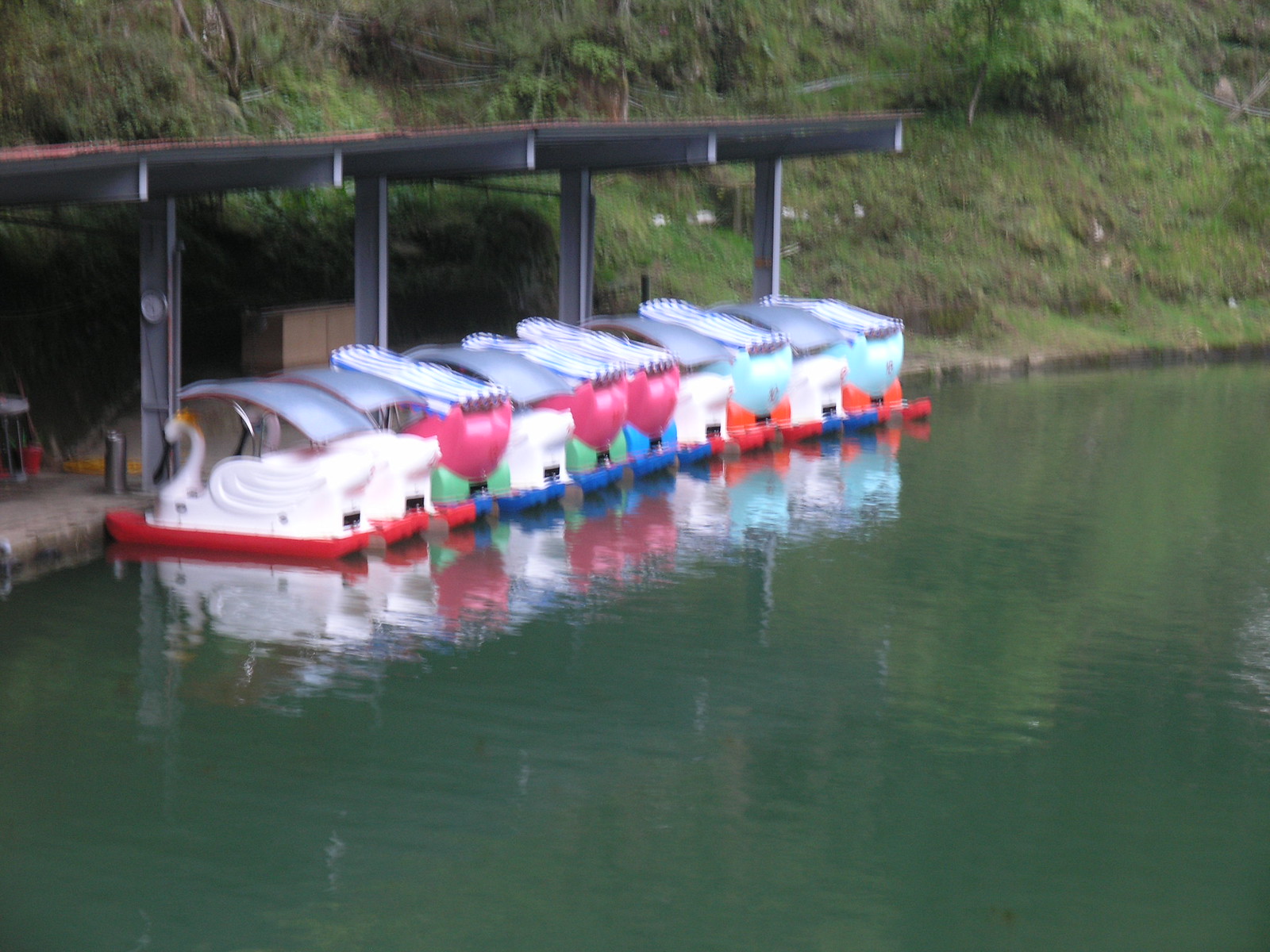In this image, we see a serene scene at a pond or lake, characterized by its calm, bluish-green water that dominates the lower portion of the background. Moored at the water's edge are a series of small, swan-shaped boats arranged in neat rows, all facing inward. The fleet includes boats of different colors: alternating between white, red, and blue swan boats, with some sporting light aqua blue and pinkish-purple accents at the back.

The swan boats feature flat, square tops providing seats and a bit of cover for riders. Toward the left, there is an open, covered walkway supported by four posts, offering access to these boats from land. Above and beyond the walkway, the upper background is lush with greenery, including grass, shrubs, and trees that adorn a gentle hillside, adding to the overall tranquil atmosphere.